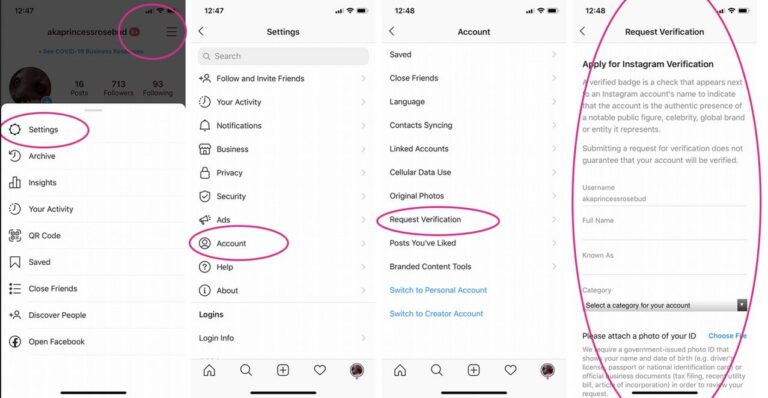A series of four smartphone screenshots are displayed side-by-side from left to right, each showing different stages and features of a social media application with a light gray background and thin white dividers between them.

**First Screenshot:**
The interface appears with a notification pop-up partially graying out the top third. The top-right corner displays standard status icons including a phone number, battery indicator, Wi-Fi symbol, and an additional unspecified icon. Beneath that, in small black text, is the username "aka Princess Rosebed." Below the username is a profile section featuring a small profile picture on the left, followed by "16 posts," "713 followers," and "93 following." The interface sports a settings option with a black icon encircled in purple. Below this, there are eight clickable options, each accompanied by an icon on the left.

**Second Screenshot:**
This screenshot focuses on the settings interface highlighted earlier. The status bar remains consistent with the first screenshot showing the time and status icons. At the top center of the screen, the word "Settings" is prominently displayed in bold. There is a search bar below this, followed by a list of seven options in black text with associated icons. The eighth option, labeled "Account," is highlighted with a purple circle. Beneath this, three more options are listed.

**Third Screenshot:**
The screen transitions to the account settings section. "Account" is now indicated at the top in place of "Settings," with the familiar seven clickable options below it. Following these options, "Request Verification" is vividly marked. The list then includes two more black-text options followed by two in blue.

**Fourth Screenshot:**
This screenshot delves into the verification request page. The header "Request Verification" stands out at the top center, framed by large vertical purple circles on both sides. Below this, the instructions "Apply for Instagram Verification" are shown. Two informative paragraphs instruct the user. Fields for submitting required details like "Username," "Full Name," "Known As," and "Category" are provided. At the bottom, there is a call-to-action requesting a photo ID, with a blue "Choose File" button for submissions followed by another paragraph explaining the details required for the verification process.